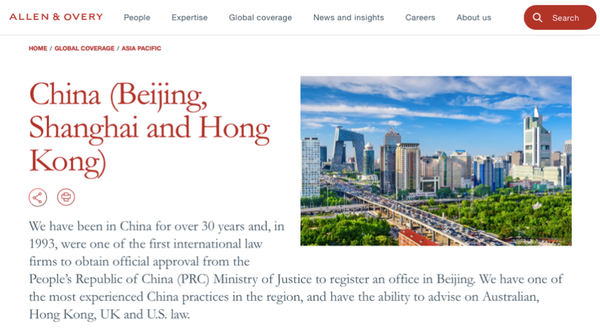This image captures the homepage of a news website belonging to Allen & Overy. The top left corner of the page prominently displays the name "Allen & Overy" in bold red letters. To the right are navigation tabs in gray reading: People, Expertise, Global Coverage, News and Insights, Careers, and About Us, ending with a red search button. 

Below the main navigation, a breadcrumb trail in smaller bold red letters guides the user through the website: Home > Global Coverage > Asia-Pacific, concluding with "China" in larger letters, followed by "Beijing, Shanghai, and Hong Kong". 

On the left, there are red Share and Print buttons. The text below them reads: "We have been in China for over 30 years. In 1993, we were one of the first international law firms to obtain official approval from the People's Republic of China (PRC) Ministry of Justice to register an office in Beijing. We have one of the most experienced China practices in the region and have the ability to advise on Australian, Hong Kong, UK, and US law."

To the right of this description is an image showcasing a skyline under blue skies with puffy white clouds. The skyline features numerous tall buildings and skyscrapers. Below the skyline, an elevated roadway with cars and verdant green trees is visible, adding a dynamic urban element to the scene.